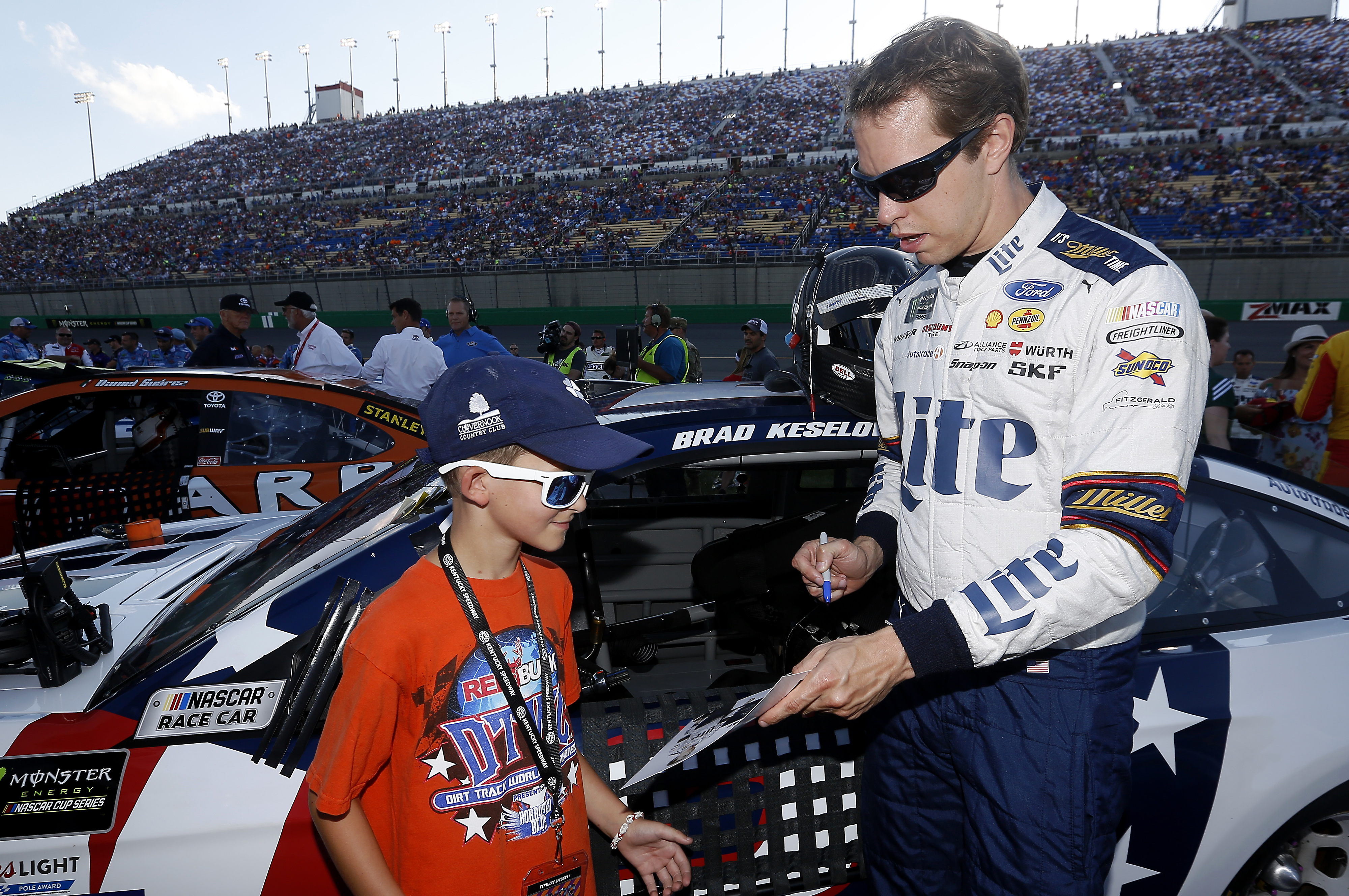Against the backdrop of a bustling NASCAR racetrack, a lively crowd fills the steeply rising bleachers under a mostly clear sky dotted with a few clouds. Tall light poles stand atop the bleachers, casting a bright light over the scene. The midground reveals the pit area with several people, some in bright yellow safety vests, attending to various tasks around the track wall. The red, white, and blue race car with a vertical blue stripe adorned with white stars and a NASCAR emblem on the left pillar stands prominently in the foreground. Before the car, a young boy, wearing a blue hat, white sunglasses, an orange shirt, and a lanyard with a name tag, beams with excitement. He holds out a book towards a race car driver clad in a white suit adorned with advertisments including “Miller Lite” and wearing dark sunglasses, who is signing an autograph. The name "Brad Keselowski" partially visible on the car behind them, hints at the driver’s identity. The scene is completed by the presence of another red race car and various advertisements, including one for Monster, decorating the surroundings.